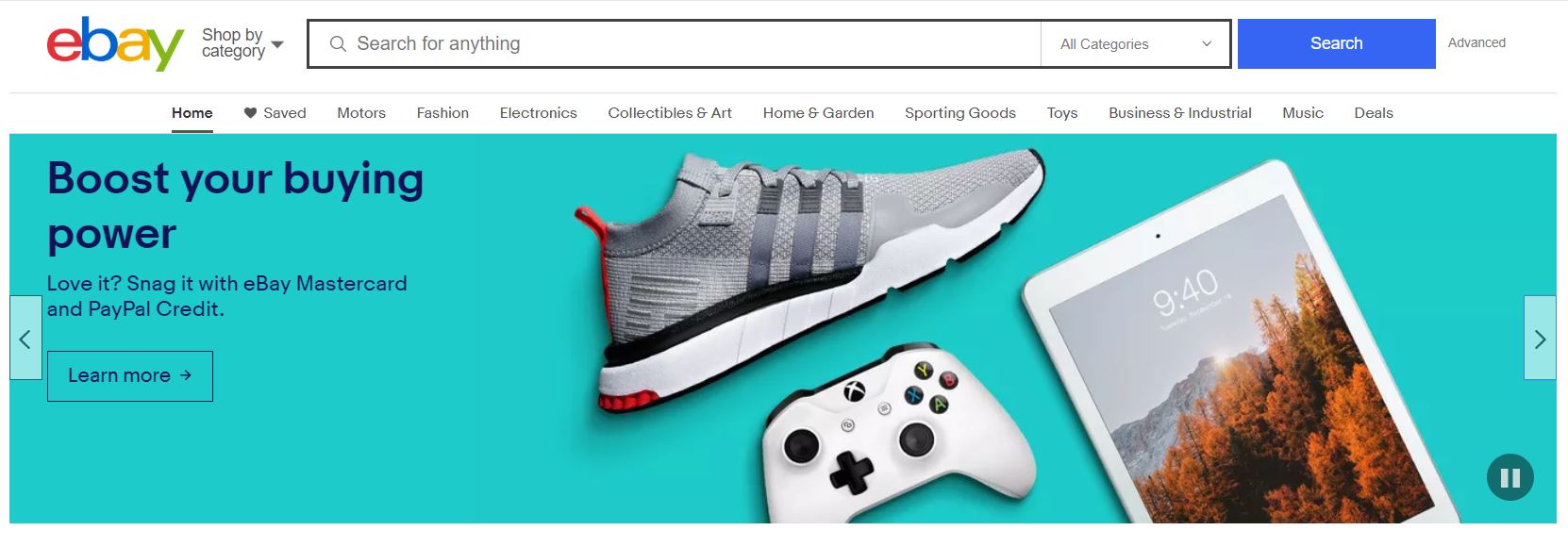This horizontally oriented image appears to be a screenshot from the eBay homepage, navigable via computer or smart device. At the very top, there's a thin gray line followed by the eBay logo in its traditional colors. Directly below this, there is a toolbar with "Shop by Category" to the left and a black-rimmed search bar featuring a magnifying glass icon and the text "Search for anything". The search bar defaults to "All Categories". Adjacent to it are a blue "Search" button and an "Advanced" button.

Below the toolbar, another thin gray line separates additional navigation options. Under this line, the highlighted and underlined word "Home" shows it's currently selected. Other categories listed include "Saved", "Motors", "Fashion", "Electronics", "Collectibles & Art", "Home & Garden", "Sporting Goods", "Toys", "Business & Industrial", "Music", and "Deals".

Beneath these options, a seafoam green section promotes eBay's financing options with the text: "Boost your buying power. Love it, snag it with eBay, MasterCard, and PayPal Credit." There is a "Learn More" button outlined for clickable interaction.

Centered within the seafoam green background are images showcasing products including a gray tennis shoe, a gaming system controller in white with black buttons, and a white tablet (possibly an iPad or Kindle) displaying a tree-filled landscape and time at the top.

Each element of this layout is meticulously designed to streamline user interaction and visually promote various products and services.